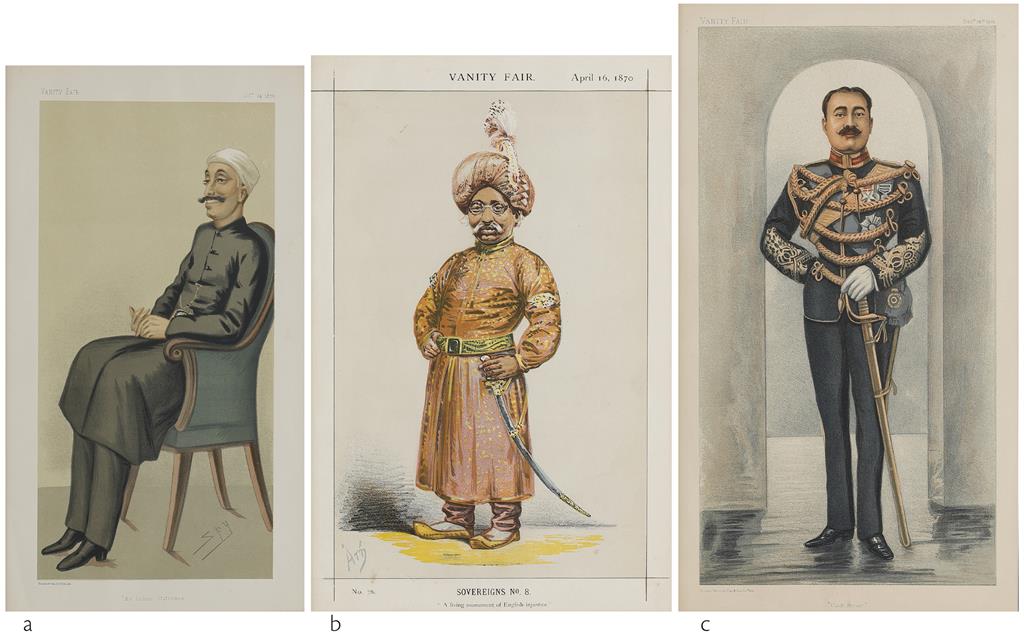This image features a plain white background showcasing three vertically oriented, vintage-style postcards, each taller than they are wide and lined up horizontally from left to right. Below each postcard, there are small lowercase alphabetical labels: 'a' on the left, 'b' in the center, and 'c' on the right. Each postcard is bordered with a light gray outline.

**Postcard 'a'** depicts a man sitting in a high-backed blue chair. He has light brown skin, a short white turban, and sports a black mustache. He is dressed in a long-sleeve black button-up tunic paired with black pants and matching boots. The background of this postcard has a light tan color.

**Postcard 'b'** showcases the cover of an issue of Vanity Fair from April 16, 1870. The headline is prominently displayed at the top. This illustration features a short man with light brown skin, wearing an elaborate brown turban. He is dressed in a long, orange tunic tied with a yellow belt at the waist. He sports pointed shoes and carries a sword. The caption under the illustration reads "Sovereign No. 8."

**Postcard 'c'** features a man with light brown skin, short black hair, and a black mustache, dressed in a distinguished black military uniform. The uniform is adorned with numerous gold braids across the chest, and he holds a long gold sword. He also wears white gloves, adding to his dignified appearance.